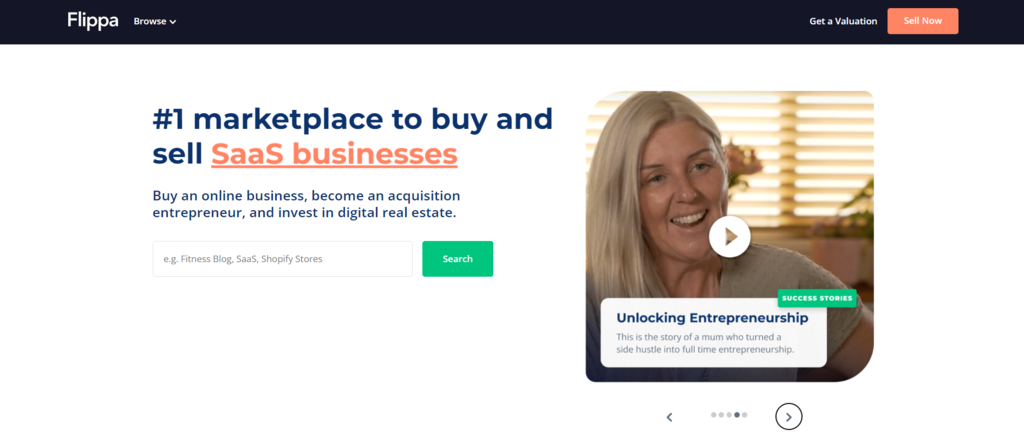This is a detailed screenshot from the company's website. At the top of the page, there's a black border approximately an inch thick. On the left side of this border, slightly inset, the text "FLIPPA" appears in large white letters. 

To the right of "FLIPPA," smaller lettering displays "Browse" accompanied by a drop-down tab. Near the right side of the black border, there's a red rectangle with the text "Sell Now" in white, and to its left, the border reads "Get a Valuation" in the same color.

Below the black border, there is a section with a white background, starting about an inch from the top and left edge. In this section, the text "£1 Marketplace to Buy and Sell" appears in blue, then follows an off-orange styled "SaaS Businesses," with the "SaaS" underlined.

Further down, blue text reads "Buy an Online Business, Become an Acquisition Entrepreneur, and Investigate in Digital Real Estate." Below this text, there is a search bar that occupies about two-thirds of the page's width, containing the placeholder text "Fitness Blog, SaaS, Shopify Stores" in black. 

Adjacent to the search bar, a green tab with the word "Search" in white can be seen.

To the right of the search bar, there's a square image of an older blonde woman, likely in her 50s. Her mouth is slightly open, showing her teeth, while she wears a brown short-sleeved shirt. Behind her, a window with blinds is visible, and a white play icon is centered over the image.

Beneath this image, a white rectangle with blue text reads "Unlocking Entrepreneurship" in bold. Below this, two lines of text explain, "how a mom turned into an entrepreneur." In the top right corner of this section, a green tab with white text reads "Success Stories."

Finally, below this, there is pagination control. A black arrow pointing to the left is followed by three grey dots, one black dot, and another three grey dots, finishing with an arrow pointing to the right encircled in black.